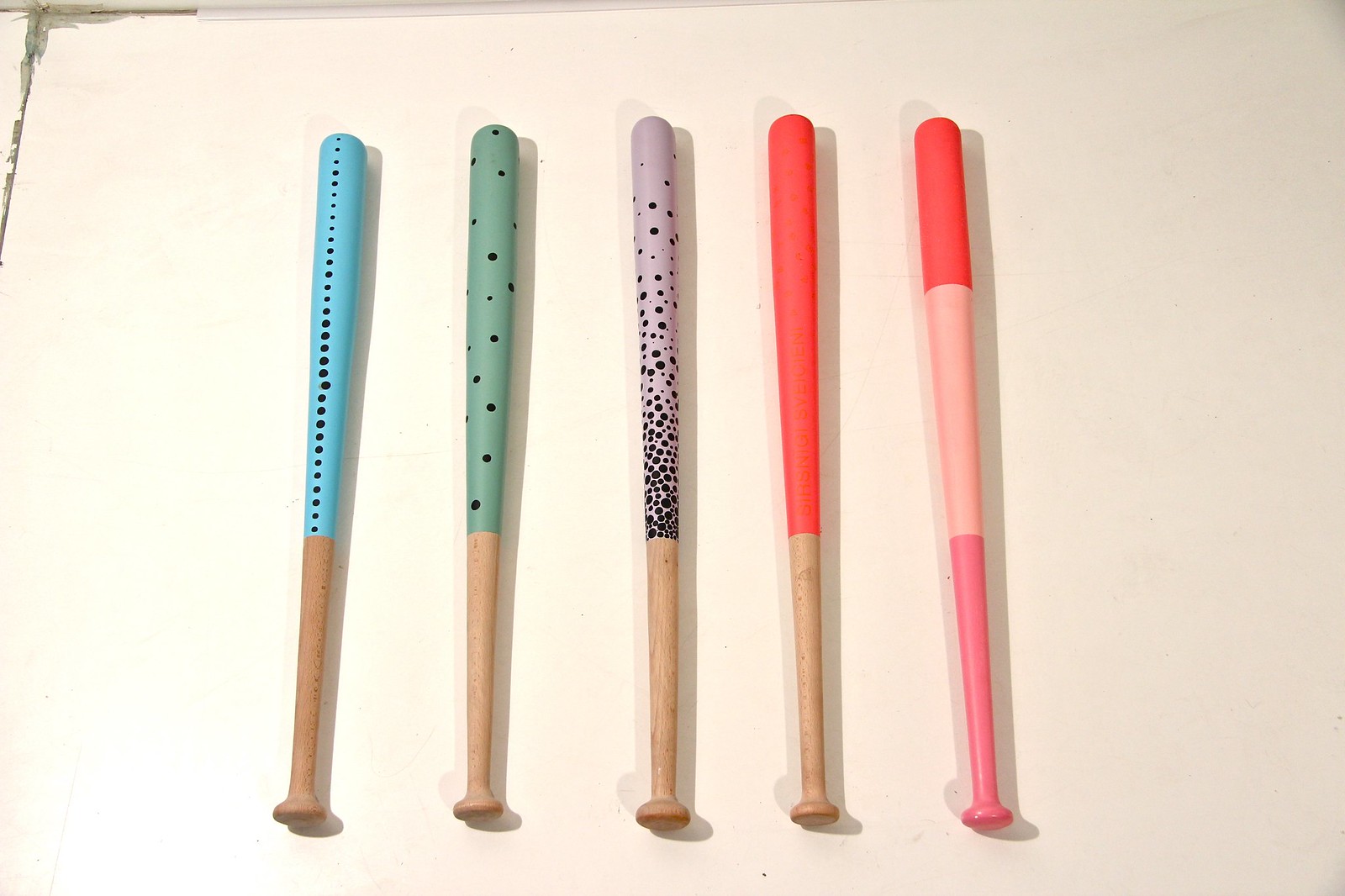This photograph captures an artistic arrangement of five wooden baseball bats, each uniquely painted and meticulously aligned against an off-white, slightly blemished background. The bats are positioned parallel to one another, spaced evenly apart, with their handles at the bottom of the image and the barrels at the top. 

The first four bats from the left maintain their natural tan wooden handles for roughly the lower third of their length. The first bat transitions to a light blue barrel adorned with a vertical line of black dots. The second features a sage green barrel sporadically dotted with black spots. The third bat's barrel is a dingy pink with densely clustered black dots at the transition, becoming more dispersed upwards. The fourth bat stands out with a solid red barrel devoid of any additional markings.

The fifth and final bat deviates from the others with a completely painted handle starting at a light pink base, transitioning to a white middle section which allows the pink to subtly shine through, and culminating in a bright red top. The entire composition is set against a white background that features gray smudges and a noticeable crack in the upper left corner, adding texture and contrast to the clean-lined arrangement of the vibrant baseball bats.